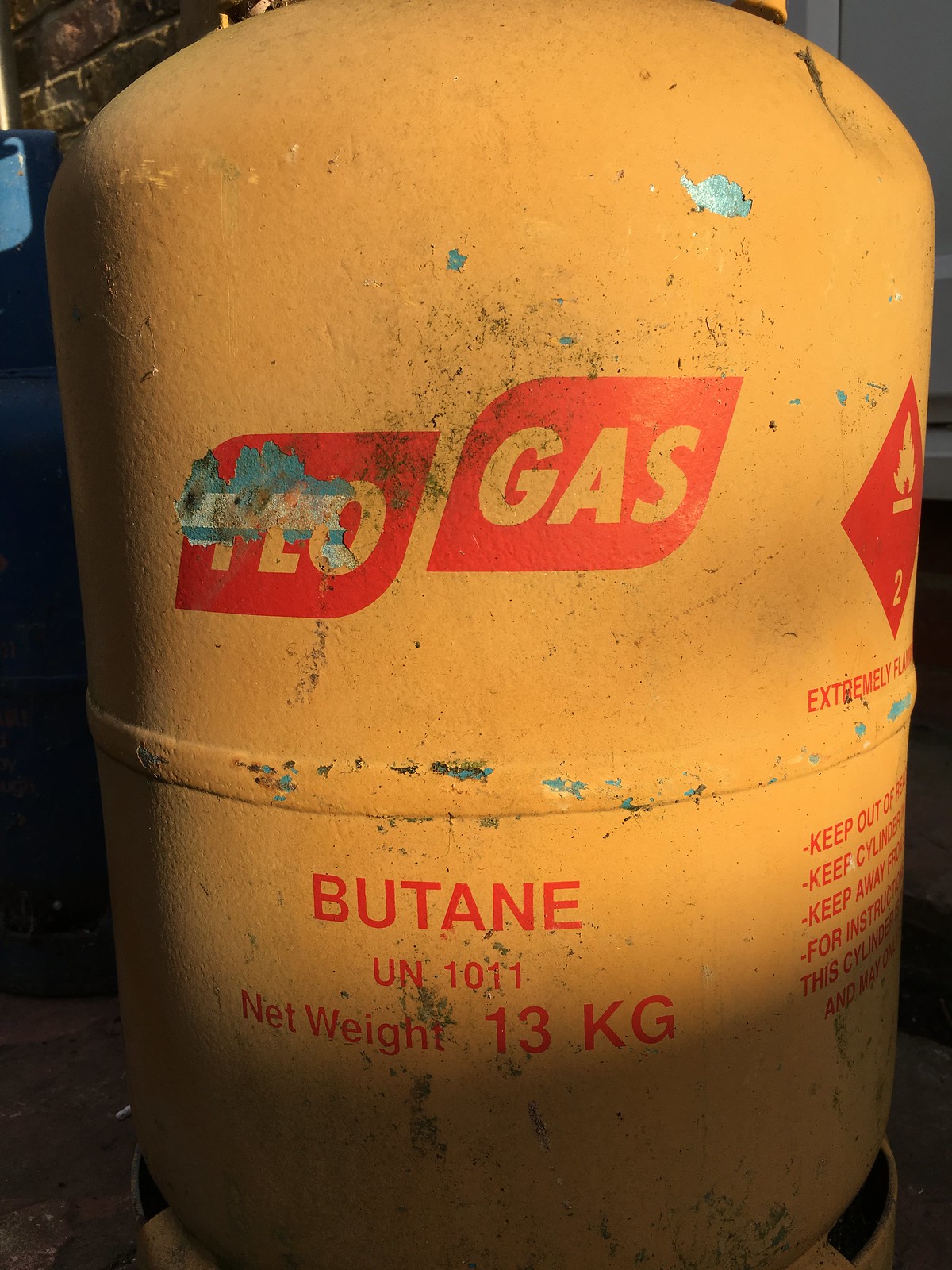This is a close-up image of a large, yellow, metal gas canister with a slightly rounded top and a flat bottom. The canister, which is mounted on a round metal structure, has faded and chipped yellow paint, revealing the silver metal beneath in some areas, particularly near its shoulder. Dominating the center of the canister is a red, leaf-shaped logo with gold text reading "TLO Gas." Below this, another red section contains text in red letters stating "Butane" and "UN 1011" followed by "Net Weight 13 kg." On the right side of the canister, there is a prominent red warning symbol indicating that the contents are "Extremely Flammable." Amid various handling instructions partially obscured along the side, warnings such as "Keep out of reach of children" and "Keep away from" can be deciphered. The canister sits under sunlight, which illuminates its upper half and part of the lower half, while the bottom is in shadow. The background includes a brown wall on the upper right and a blue barrel on the left. The overall condition of the tank appears worn and somewhat dirty.